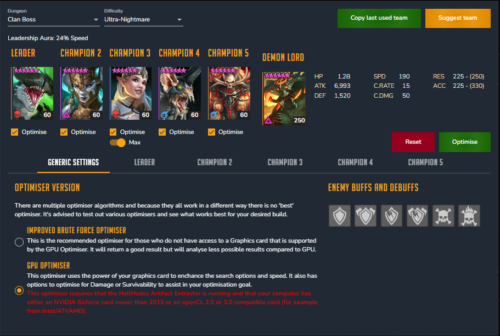The image is a detailed screenshot of a webpage, characterized by a blue background. At the top, there are six cartoon character avatars labeled with titles such as "Leader," "Champion Two," "Champion Three," "Champion Four," "Champion Five," and "Champion." Below these avatars appear to be scoring levels indicated by text in orange and white, though the exact details are too small to discern clearly. 

In the top right corner, there are green and orange buttons, likely for navigation or interaction, though the specific labels on these buttons are not legible. Along the bottom right side of the image, there are sections labeled "Enemy" and "Benefits," possibly indicating some comparative or informational elements.

Additionally, there are clickable white icons present, although their functions remain unclear. The red and green buttons scattered throughout the screenshot might indicate options or actions, but again, the exact wording is unreadable due to image size.